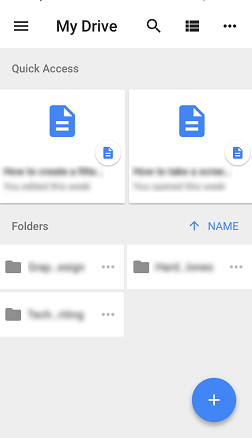The image appears to be a screenshot from the Google Drive app or website interface, showcasing several distinct UI elements. At the top left corner, there's a hamburger menu depicted as three horizontal black bars. To its immediate right, the text "My Drive" is displayed in black. On the top right corner, three icons are visible: the first icon is a magnifying glass, followed by an icon resembling books stacked together, and lastly, three vertically aligned black dots.

Directly below these icons is the label "Quick Access" placed on the far left. Underneath "Quick Access," there are two sections with text that is intentionally blurred out, with the first section featuring a blue document. 

Further down, there is a "Folders" section containing three folders—two positioned on the left side and one on the right side. At the very bottom right of the image, a blue circle with a white plus sign is noticeable. The areas to the left and above this plus symbol are empty. The overall background color of the interface is light gray, while the interior of each section and folder thumbnail has a pure white background.